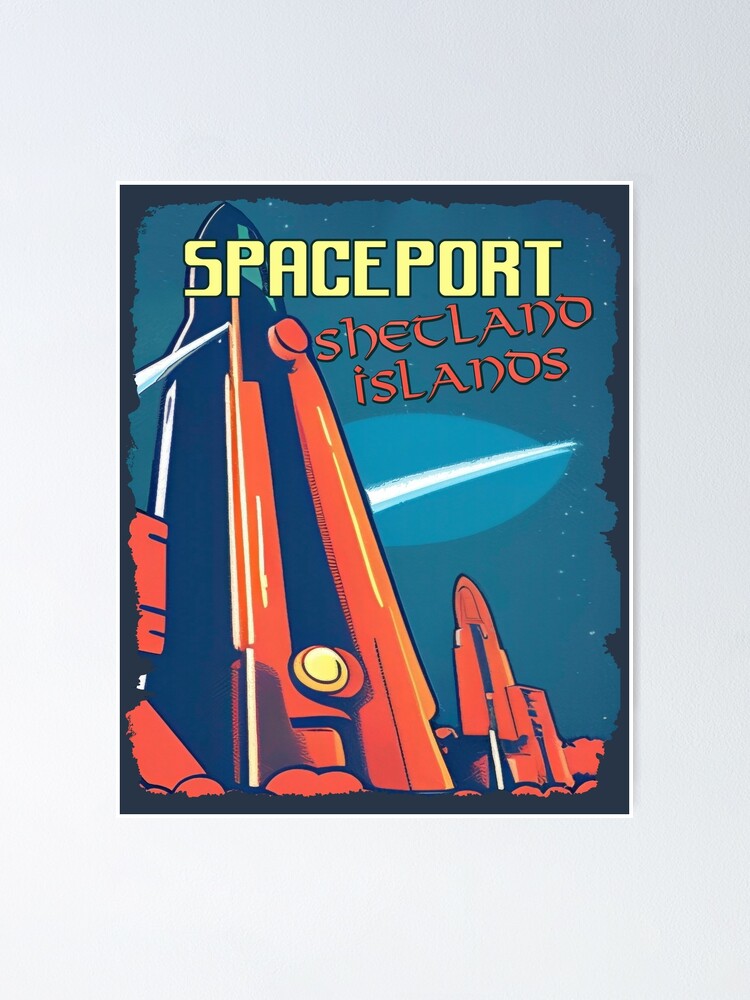The image is a stylized comic book cover illustration with a thick, irregular black border surrounded by a white frame. At the top, bold yellow capital letters read "SPACEPORT," while directly below, in a different font and a matching orange hue to the depicted rockets, the text reads "Shetland Islands." The central illustration features two large red rockets—one prominent and tall, with the other slightly smaller and positioned to the left—each adorned with yellow and white detailing. The background showcases a dark blue, star-filled sky, dotted with white stars and the faint trail of a comet streaking through the scene, providing a celestial atmosphere. The entire poster, reminiscent of a retro advertisement, vividly illustrates a futuristic launch site against the serene cosmic backdrop.